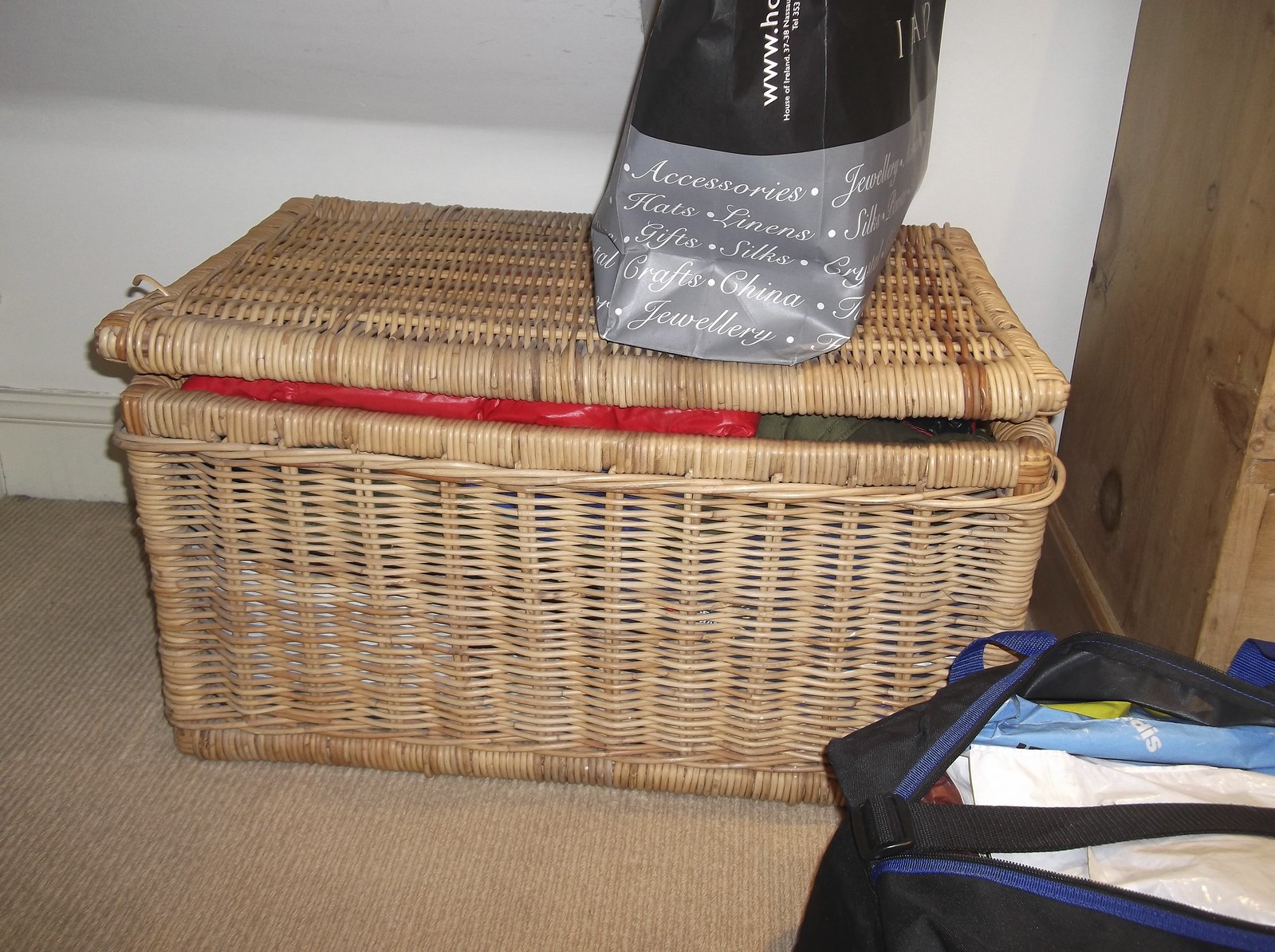The photograph features a large wicker basket, constructed from light brown bamboo wood, resembling the size of a footlocker. The basket is so full that its lid cannot close completely, revealing a red object and hints of dark olive green within. Draped over the wicker basket is a shopping bag, characterized by a black upper half and a gray lower half. The gray portion is inscribed in white with various words: accessories, hats, linens, jewelry, gifts, silks, crafts, and china. This inscription appears on all sides of the bag. 

In the bottom left corner, an open black duffel bag with blue fabric handles and blue lining around the zipper is visible. Inside this duffel bag, partly obscured, is a white plastic bag and a blue plastic bag that bears the partially visible letters "S.I.P."

The scene is set against a backdrop of a white wall, with a portion of a brown wooden shelf or pillar visible in the right-hand corner. The flooring below is covered with a light brown or beige fabric, adding to the overall intricacy and texture of the composition.